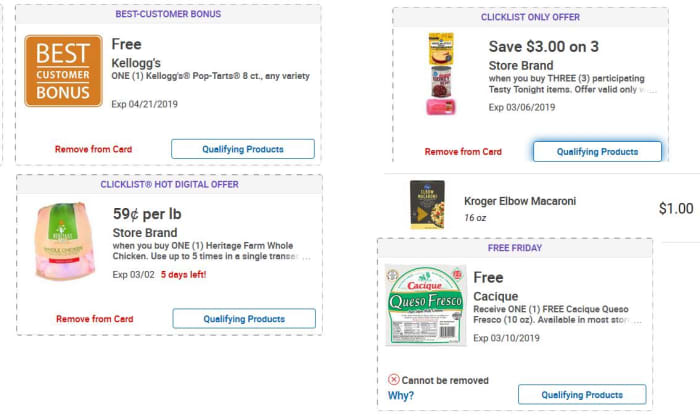The image displays a collection of digital coupons, presumably within an online platform, but it is unclear whether it is a website or an app. The coupons are visually distinguished by a perforation design, simulating the look of traditional paper coupons. 

1. **Free Kellogg's Pop-Tarts (8 count, any variety)**: This coupon offers a free pack of Kellogg's Pop-Tarts with any variety consisting of 8 counts.
2. **Save $3 on Three Participating Tasty Tonight Items**: This coupon provides a $3 discount when you purchase three items from the Tasty Tonight range.
3. **59¢ per Pound for Heritage Farm Whole Chicken**: This coupon provides a deal where Heritage Farm whole chicken is priced at 59 cents per pound.
4. **Free Cacique Cheese**: This coupon offers a free item of Cacique cheese, though the pronunciation is noted as uncertain.

Beneath each coupon, there are interactive links such as "Remove from card" and "Qualifying products". Additionally, there is a smaller coupon positioned among the others, offering **Kroger Elbow Macaroni for $1**.

This detailed layout suggests a user-friendly interface for managing and redeeming digital savings.